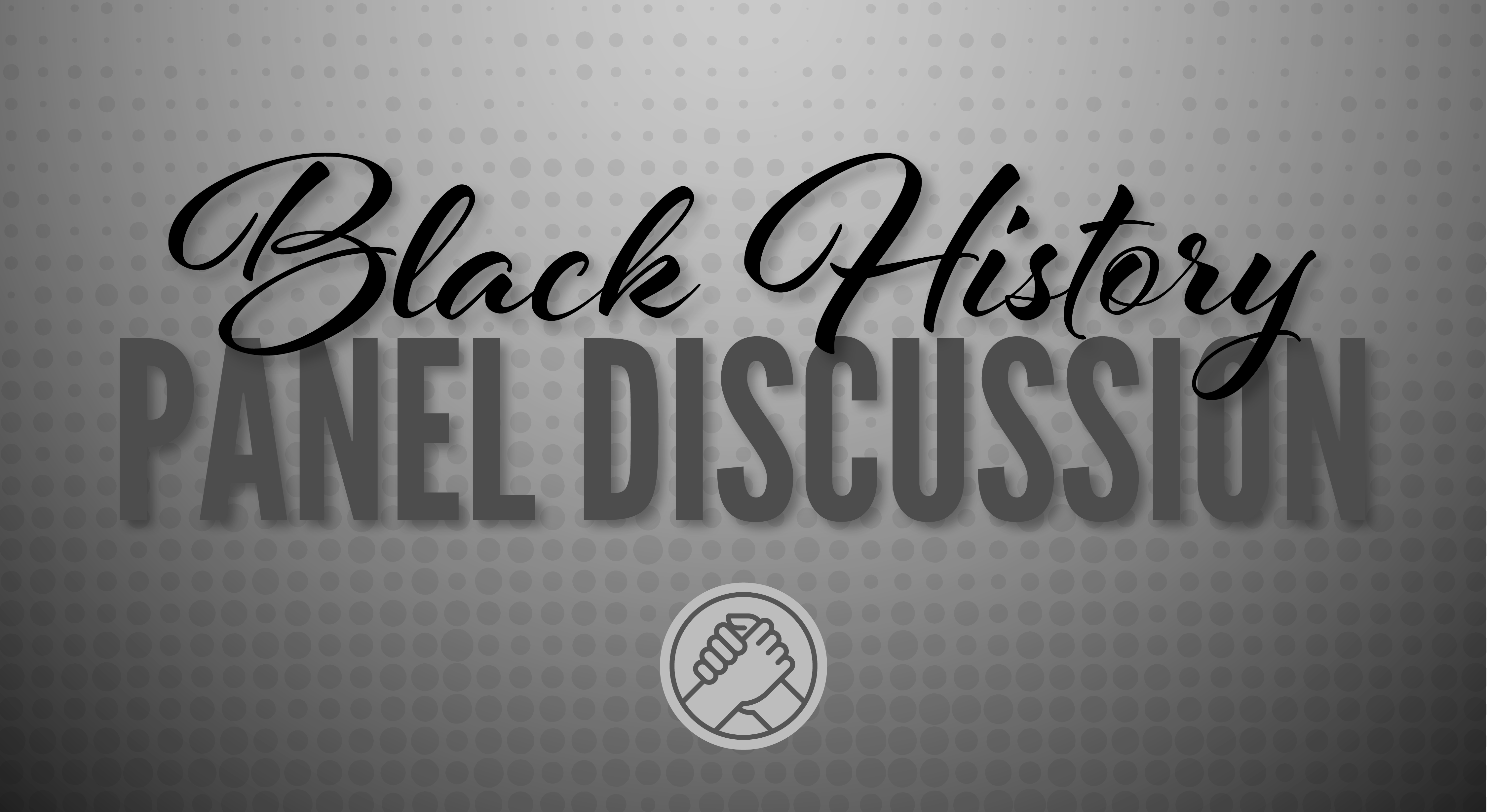The grayscale image features a gradient gray background with a pattern of circles that transition from a regular arrangement at the bottom to an irregular, fading pattern at the top. Central to the image, there is a light gray circle with a dark gray outline, inside which two hands, depicted as outlined figures, clasp each other, symbolizing solidarity. Above this emblem, in the very center of the frame, two lines of text are prominently displayed. The top line in sharp, black cursive reads "Black History," overlapping slightly with the blocky, dark gray sans-serif text below that says "Panel Discussion." The background’s gradient shifts from light gray at the top to a darker shade at the bottom, enhancing the dynamic design of the image.